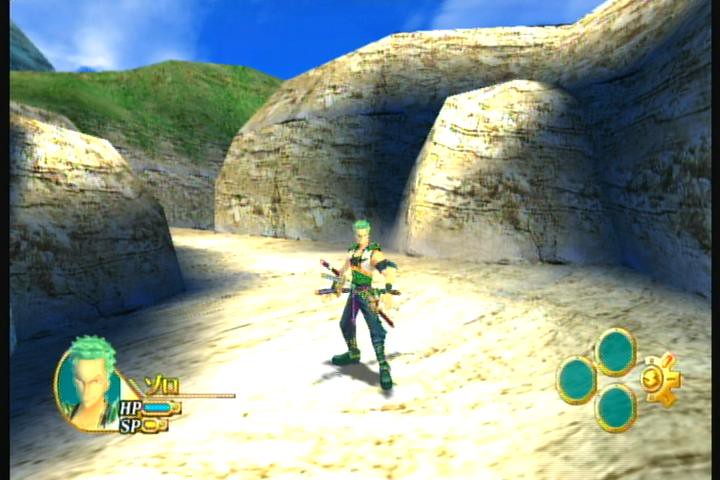This detailed screenshot captures a scene from an old-school, retro fighting game, reminiscent of titles like Mortal Kombat. The central character, a distinctive figure with bright green hair and adorned in green dungarees and a white shirt with green shoulder pads, stands amidst large boulders, one of which is covered in grass. The peaceful blue sky peeks through the rocky backdrop, adding a touch of serenity to the scene. The character, who appears equipped with two crossed swords tucked into his belt, radiates a vibe that ties into his color theme—predominantly green. His in-game representation includes a pointy face and matching green hair, visible in the bottom-left corner of the screen alongside his HP (displayed with a green bar) and SP (yellow bar) meters. Additionally, three circles with green centers and yellow outlines, accompanied by semi-shield icons, are aligned on the right side. The overall image, possibly captured from a TV screen, introduces viewers to this intriguing character in an iconic, nostalgic gaming moment.